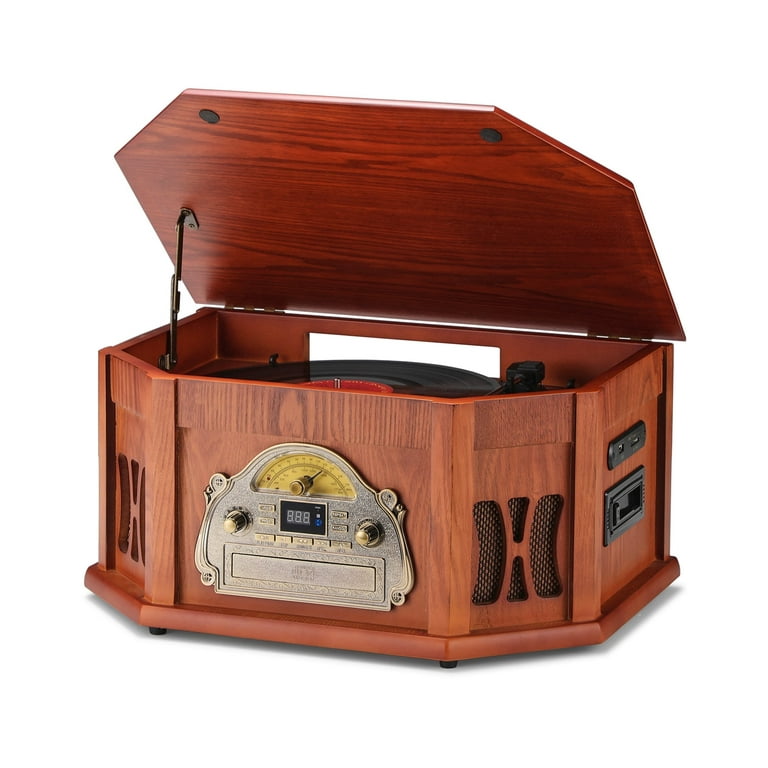This image captures a vintage-style record player housed in a wooden box made of cherry wood, giving it a classic and elegant appearance. The record player’s lid is open, revealing a 33-size black vinyl record with a distinctive red rim around its center seated on the turntable. Flanking the front of the box are two speakers, while a metal plating adorns the box’s center front with two knobs and an old-fashioned silver gauge, likely for volume and sound control. The gauge displays digital numbers reading “888” along with a yellow, analog dial. On the right side of the box, there are input ports and possibly a handle. The craftsmanship of the record player, combined with its functional dials and inputs, gives it an air of nostalgic sophistication.